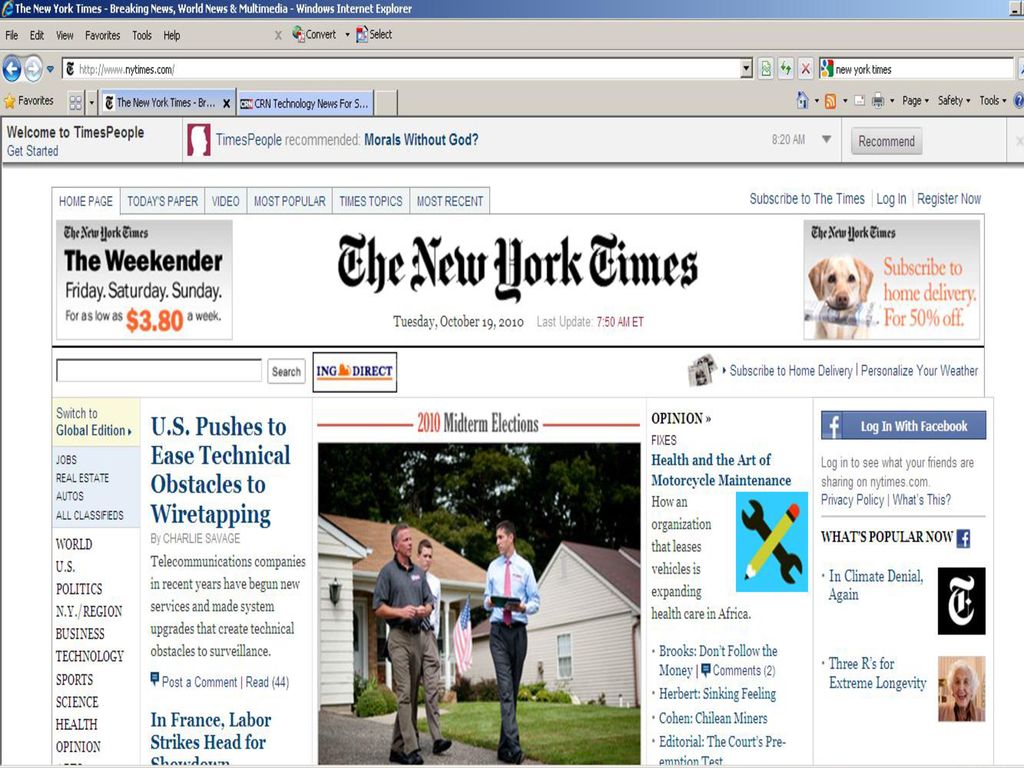This image is a nostalgic screenshot of the New York Times website, reflecting an older internet era or device interface. At the top left, the search bar prominently displays NewYorkTimes.com, accompanied by a blue back arrow. Centered on the screen is a promotional tab for the New York Times Weekender, offering Friday, Saturday, and Sunday editions for as low as $3.80 a week, with the price prominently highlighted in orange text.

To the right, there's an endearing image of a yellow labrador retriever holding a newspaper in its mouth. Adjacent to the dog image, bold orange text advertises a 50% discount for subscribing to home delivery.

Beneath this, various headlines capture attention. One headline reads: "U.S. Pushes to Ease Technical Obstacles to Wiretapping," detailing how recent service updates and system upgrades by telecommunication companies have created barriers to surveillance. Readers are invited to post a comment or view the 44 existing comments through a clickable blue link.

Another headline, "In France, Labor Strikers Head for Showdown," indicates rising tensions. 

On the right side, some opinion pieces are noted, including one intriguingly titled "Health and the Art of Motorcycle Maintenance," symbolized by a wrench and a pencil logo.